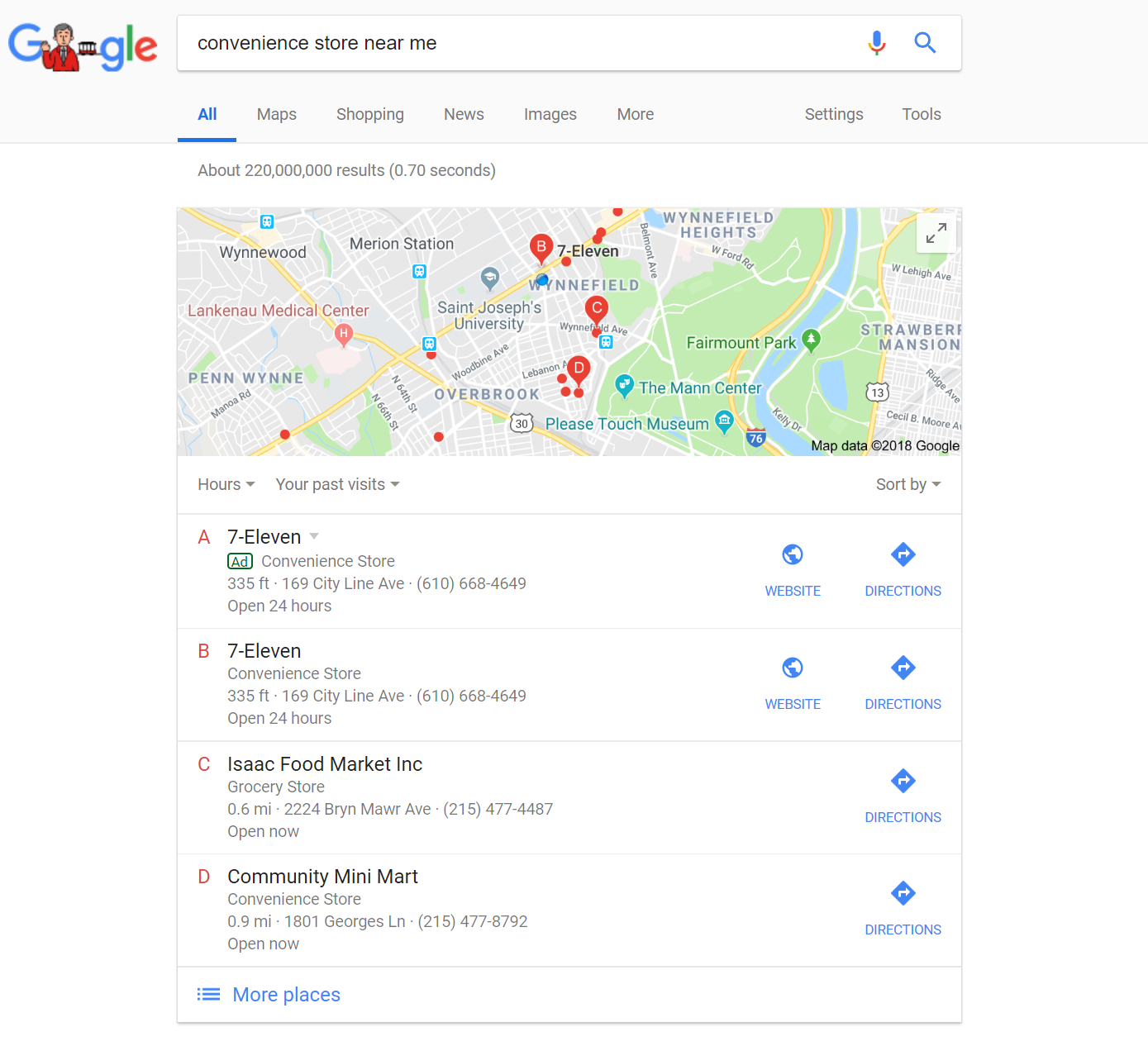The image depicts a Google search results page, featuring a sleek gray bar at the top. On the top left, the Google logo is creatively illustrated: the first 'O' includes a man in a red suit, while the second 'O' resembles a trolley car.

Centered below the logo, the search bar contains a query for "convenience store near me." Directly beneath this, the navigation menu displays options such as 'All,' 'Maps,' 'Shopping,' 'News,' 'Images,' 'More,' 'Settings,' and 'Tools,' with the 'All' tab currently selected. The search has generated approximately 220 million results in 0.70 seconds.

A prominent rectangular map dominates the middle of the page, highlighting various neighborhoods like Winfield, Overbrook, Winfield Heights, Penwyn, and Strawberry Mansion. The map features three marked locations in red.

The search results are listed below the map. The first result is an advertisement for a 7-Eleven convenience store, located 335 feet away at 169 City Line Avenue, and is open 24 hours. The second result mirrors this, also featuring the same 7-Eleven store and address. The final results, labeled 'C' and 'D,' are for 'Isaac Food Market Inc' and 'Community Mini Mart,' respectively.